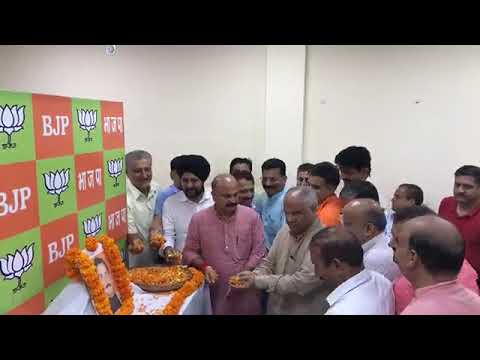This rectangular image, cropped by thick black strips at the top and bottom, captures a solemn ceremony of older Indian men, possibly of cultural or religious significance. The men are gathered around a central white table adorned with orange decorations, notably a photo frame encircled with vivid orange flowers. There's a bowl on the table holding the same type of orange flowers, further emphasizing the ritualistic or commemorative atmosphere. Situated in front of a tilted billboard with a bright orange and green checkerboard pattern, each orange square prominently displays the letters "BJP" in white, while the green squares feature a white lotus-like drawing. The background showcases a beige, light gray wall interrupted by a single column, adding depth to the image. One man standing to the right of the table has his hands clasped together, possibly in a gesture of reverence or prayer, enhancing the ceremonial scene.